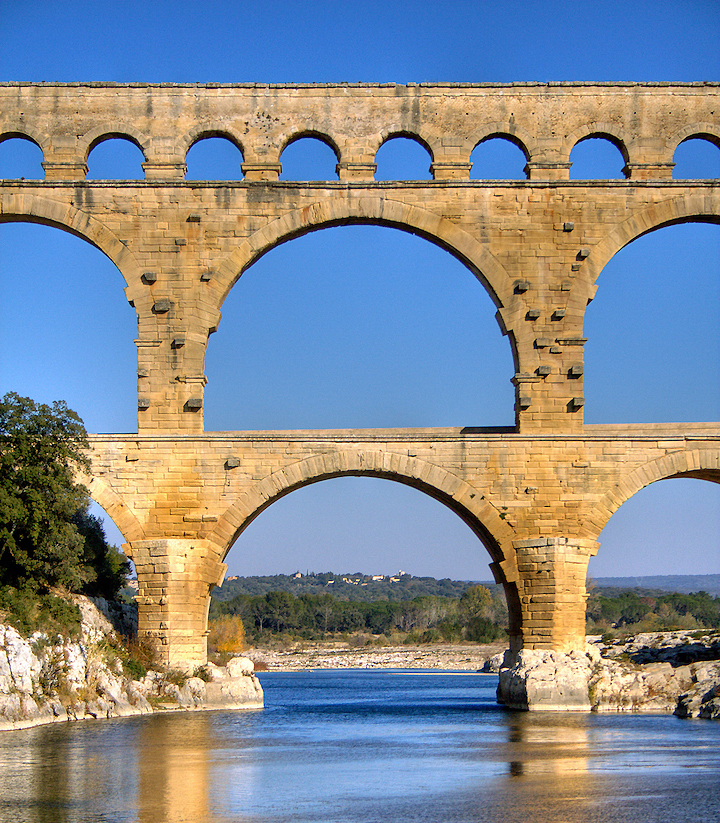The image captures an ancient stone structure resembling the Pont du Gard aqueduct. This imposing bridge, likely built around 2,000 years ago, features multiple tiers of arches crafted from meticulously stacked stone blocks. The aqueduct spans over a serene stream or river, with its rocky shores dotted by greenery. Trees flank the ancient edifice, and in the distant background, a cityscape nestled in the hills suggests a setting akin to Los Angeles. The construction includes arches upon arches, creating a mesmerizing pattern that may have once supported water flow or passage but now appears primarily decorative. Despite its age, the structure remains in remarkably good condition, possibly restored in the past, with protruding stones hinting at its historical complexity.